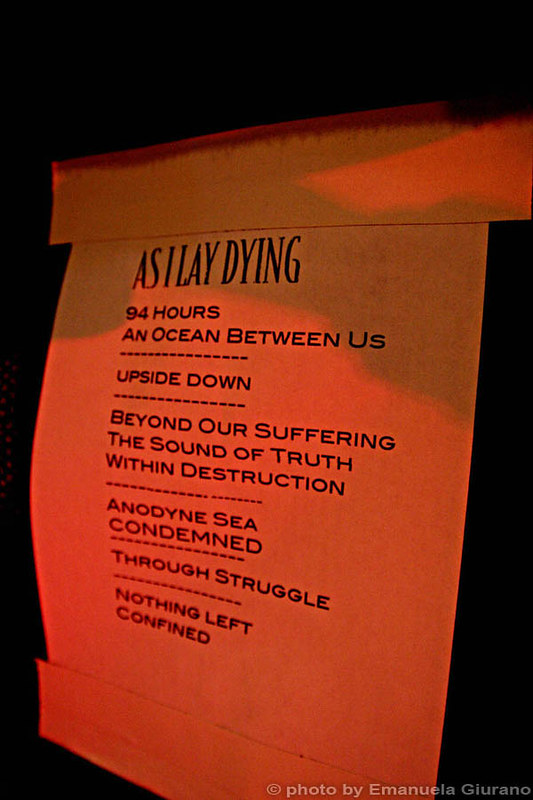The image depicts a set list for the band "As I Lay Dying," typed on a piece of white printer paper. The paper is affixed to a dark, indiscernible surface with two very thick pieces of tape, one at the top and one at the bottom. The text on the paper lists a series of song titles in black font. At the top, the band name "As I Lay Dying" is prominently displayed in a tall font, followed by the song titles in a shorter all-caps font: "94 Hours," "An Ocean Between Us," "Upside Down," "Beyond Our Suffering," "The Sound of Truth," "Within Destruction," "Anodyne Sea," "Condemned," "Through Struggle," "Nothing Left," and "Confined." Dotted horizontal lines separate some of the titles. The image appears to be illuminated by an orange or red light, giving the paper a tinged hue. A watermark at the bottom right of the paper reads, "Photo by Emanuela Giurano."